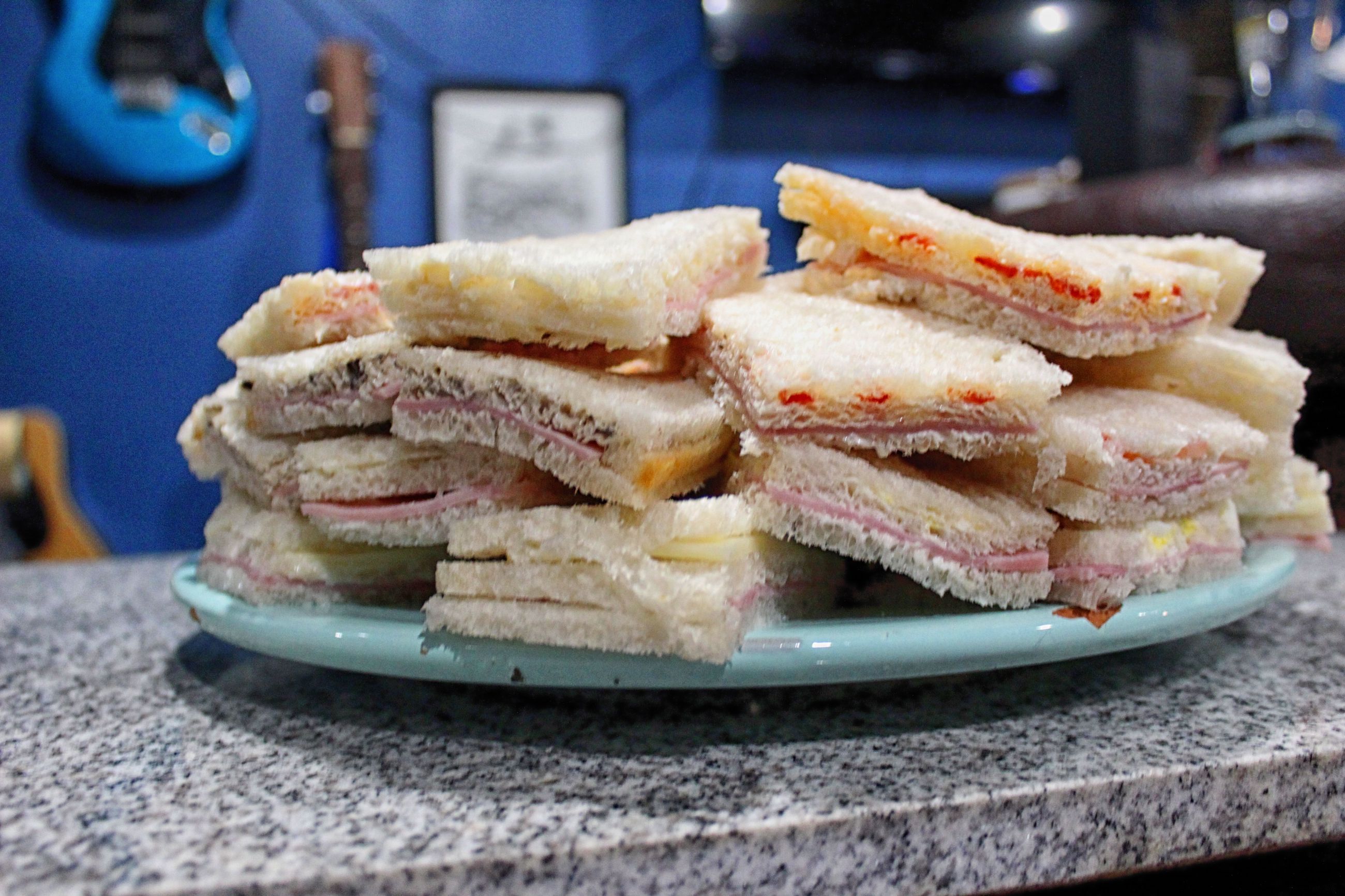The image showcases a sky-blue round plate, slightly chipped around the rim, positioned on a white granite countertop speckled with black. The plate is piled with crustless sandwiches made from thin white bread, filled with bits of ham and possibly pimento cheese, with some containing small red pieces that resemble peppers. The sandwiches appear somewhat limp and are stacked haphazardly. In the blurred background, a blue wall adorned with at least three guitars can be seen on the left side, with one blue and black guitar, one brown and black guitar, and just the top of another guitar partially visible. On the upper right side of the background, a brown leather couch and a black ceiling with white lights are also discernible.